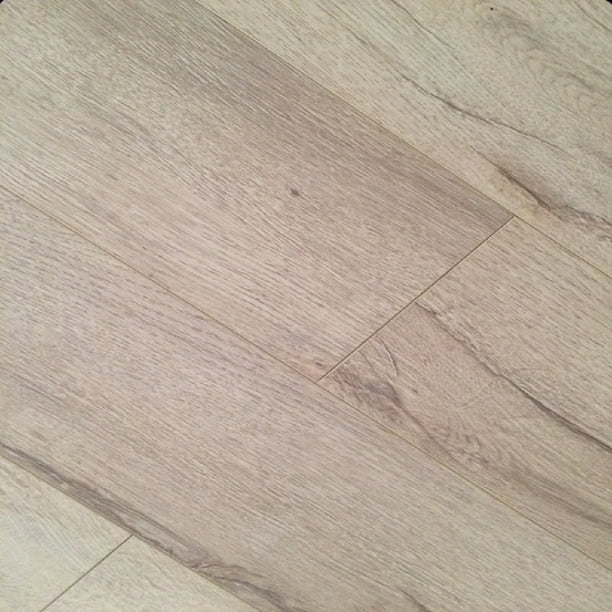The image captures a close-up of a tan, synthetic wood floor with a simulated wood grain pattern. The flooring consists of six visible pieces, with two long joints and three shorter joints connecting the pieces. The boards, installed diagonally, exhibit variations in the wood grain and color, featuring shades of tan, beige, and darker brown, with slight hints of gray and red. Some planks also showcase darker and lighter highlights. Although primarily smooth, the flooring appears to have a slight texture upon touch. This detailed view emphasizes the interconnectedness and alignment of the individual pieces, filling the entire frame without any additional text or context, suggesting it's an interior floor, likely used in rooms such as kitchens or entryways.